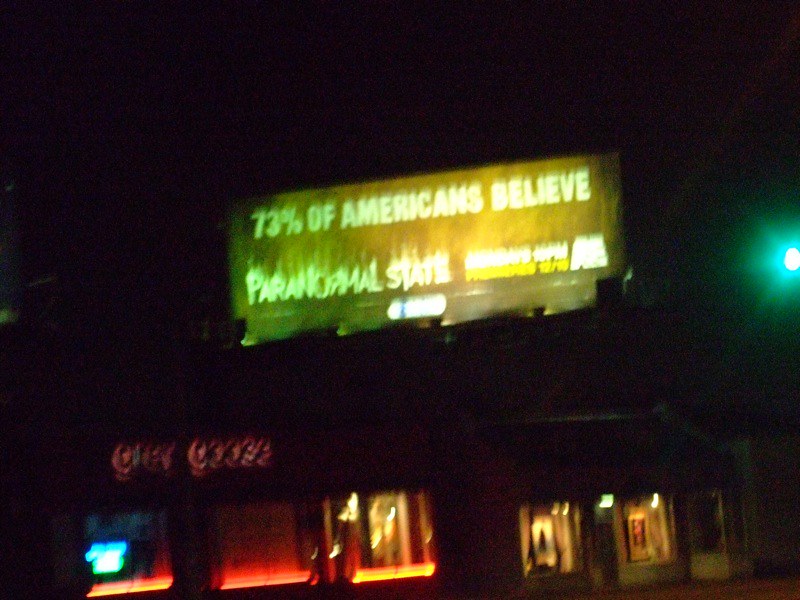This is a blurry night-time photograph dominated by a fluorescent billboard in the center. The sign, glowing in varying shades of green and yellow neon lights, reads "73% of Americans believe paranormal" with some illegible text following. The sky in the background is completely black, adding to the overall darkness of the image. To the right, a bright street light emits a blue-green hue. Below the billboard, there appear to be storefronts with mixed amber and red lighting, with one possibly displaying the word "Goose" in red neon. The image lacks any visible people, animals, plants, or vehicles, maintaining a focus on the illuminated sign and the shadowy structures below it.